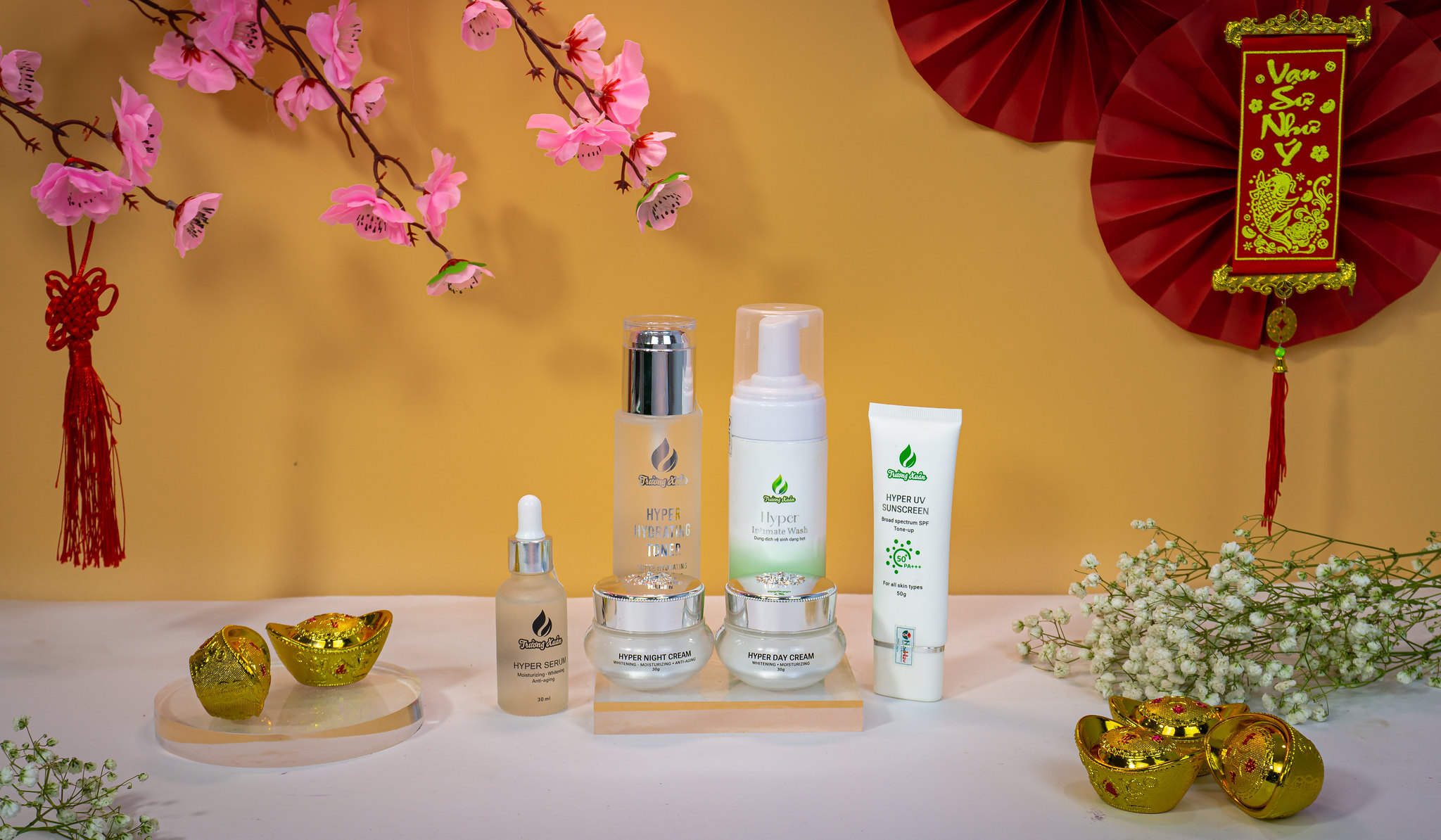The image presents an elegantly arranged skincare product display set against a vibrant yellow backdrop. On the table, six distinct items are lined up meticulously: four bottles and two jars. From left to right, the bottles include a 'Hyper Serum' emphasizing moisturizing and anti-aging properties, a 'Hyper Hydrating Toner', a 'Hyper Wash', and another indistinct wash product. The final bottle on the right showcases 'Hyper UV Sunscreen' with a sun protection factor of 50 PA+++. The two accompanying jars are labeled 'Hyper Night Cream' and 'Hyper Day Cream' respectively. Enhancing the aesthetic, sprigs of delicate baby’s breath lie gracefully alongside the products. The background features a rich yellow wall adorned with a few flowers emerging from the left side. In the upper right corner, two striking red circular fans appear, each intersected by banners inscribed in an unidentifiable language, adding an exotic flair to the overall composition.